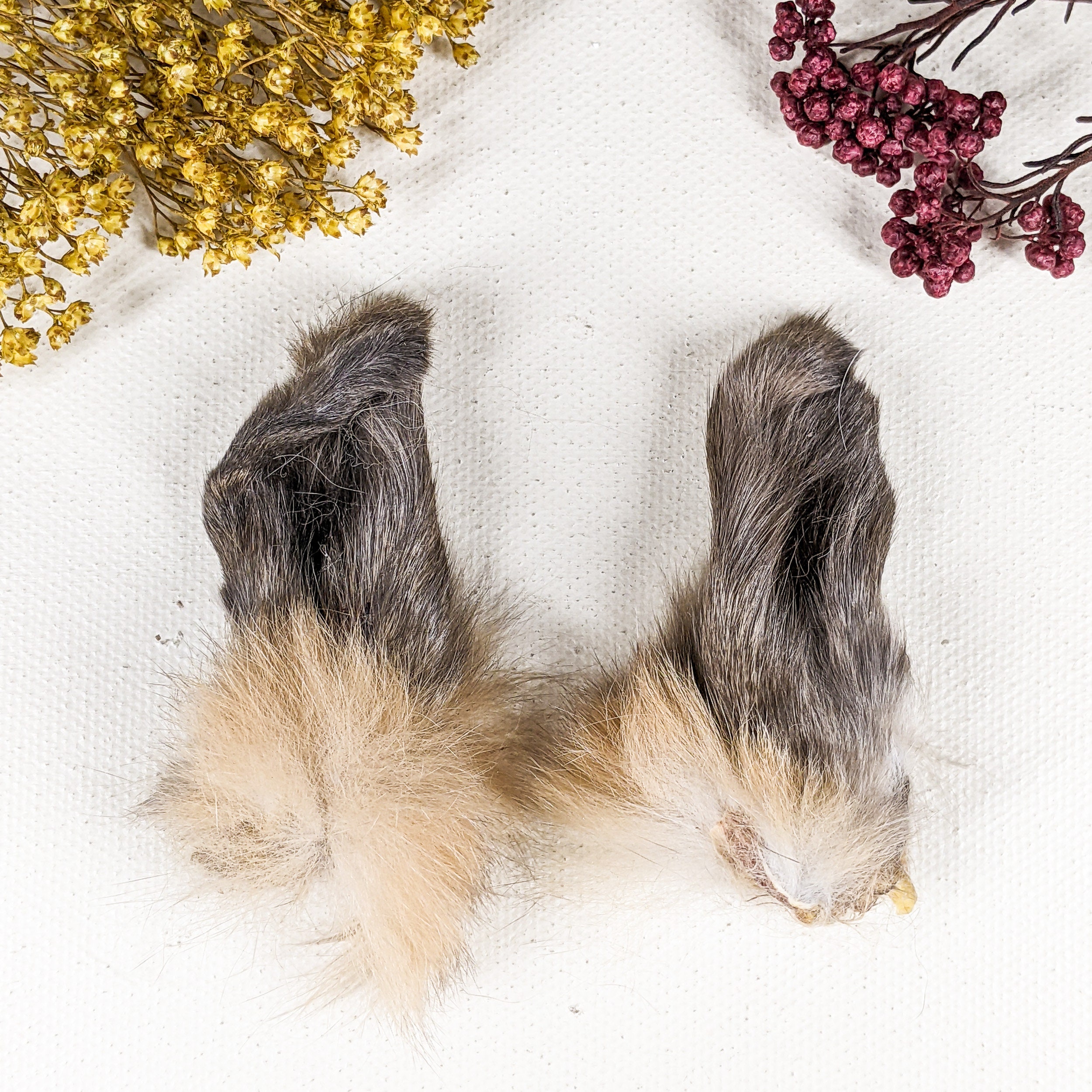The image showcases a neatly arranged display set against a white fabric background. In the center, two animal ears, with gray and light brown fur forming a U-shape, draw immediate attention. These ears exhibit a gradient of colors with gray at the tips transitioning to a lighter tan towards their bases. The placement and texture suggest they might belong to a dog or bunny, though no body is visible. Complementing the ears, a vibrant contrast of dried flowers frames the scene; yellow flowers elegantly protrude from the upper left corner, while deep burgundy red flowers, possibly dried berries, extend from the upper right. Shadows cast by the objects add depth, though they appear inconsistent across the image. The overall composition exudes a thoughtful yet slightly eerie display, combining organic textures and rich colors against the soft, clean backdrop of the white fabric.